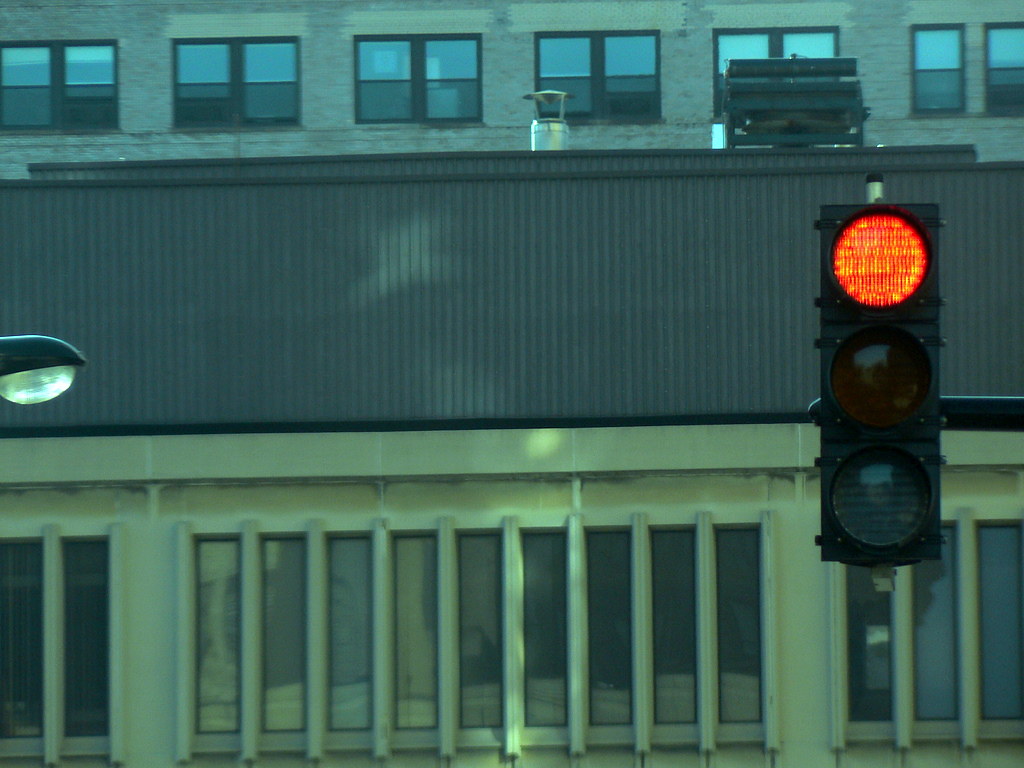This outdoor photograph captures a scene dominated by a tall building in the background. Positioned prominently on the far right-hand side of the image is a traffic light facing directly forward. The red light at the top is lit, while the yellow and green lights below it are unlit, with the yellow light appearing almost black. On the far left side of the image, a street light is partially visible; only the oval-shaped bottom half is illuminated, leaving the top half in shadow.

The upper portion of the building's facade features six rectangular windows, each divided into four smaller panes. Below these windows, a grey-colored awning extends across, providing some shading. Beneath the awning, there are barred windows, contributing to a sense of security or restriction. The building itself has a warmer, yellow-toned exterior on the lower levels, contrasting with the cooler, grey-toned upper windows. The composition of the image balances the imposing structure with urban details, capturing a moment of city life under a regulated red light.